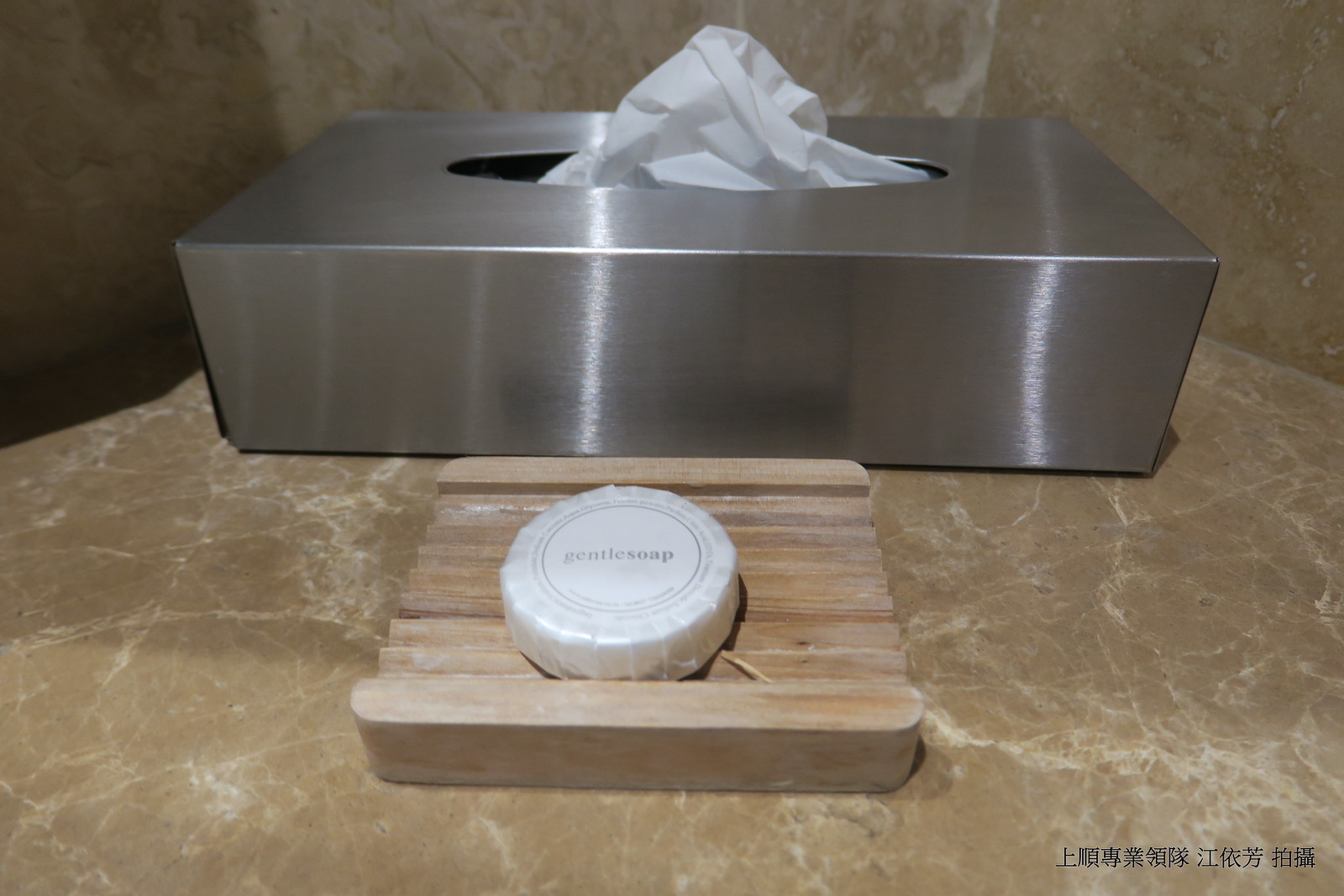In this photograph, we see a meticulously designed bathroom countertop adorned with elements of subtle luxury. The surface and walls are covered in a marbled finish, characterized by a rich brownish-yellow or dark gold hue interlaced with thin white veins that lend an intricate and elegant pattern. At the bottom right corner of the countertop, black Asian characters are visible, adding an element of cultural sophistication.

In the background, a sleek, silver metal tissue box stands prominently. Its long rectangular form is complemented by a neatly folded white tissue emerging from the slot, creating a triangular shape. Positioned in front of the tissue box is a wooden soap holder, notable for its crafted ridges that support its functionality and aesthetic appeal. Centered within the holder lies a circular bar of soap, wrapped and textured to perfection. The soap features gray text that reads "Gentle Soap," underscoring its intended use and delicate nature. Together, these elements create an ambiance of refined elegance and practical grace in what appears to be a beautifully appointed bathroom space.